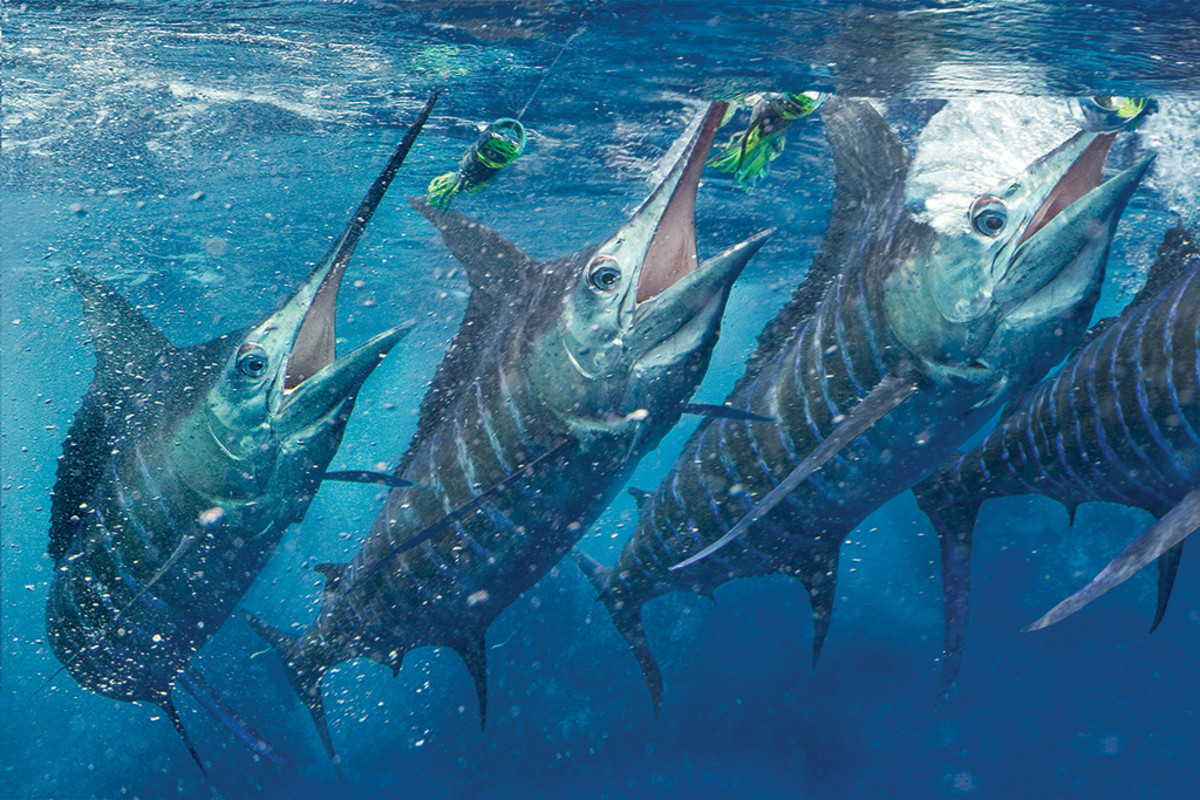This underwater photograph captures a dynamic scene featuring four swordfish, each in the midst of breaching the water's surface. All four fish are uniformly striped with dark blue and light blue bands, and their large, prominent dorsal fins create a striking visual. The identifiable sword-like noses, ranging from 10 to 12 inches in length, are indicative of swordfish, and three are clearly visible breaching upwards, with the remaining fish partially obscured, showing only the back half of its body but mimicking the same movement. The swordfish appear to be responding to bait placed by the photographer, a detail emphasized by their open mouths and the visible eyes fixed on their target. The scene is accented by bubbling water, emphasizing the rapid motion and energy of the fish as they approach the surface. The shimmering silver of their scales adds a final touch of brilliance to this captivating marine moment.